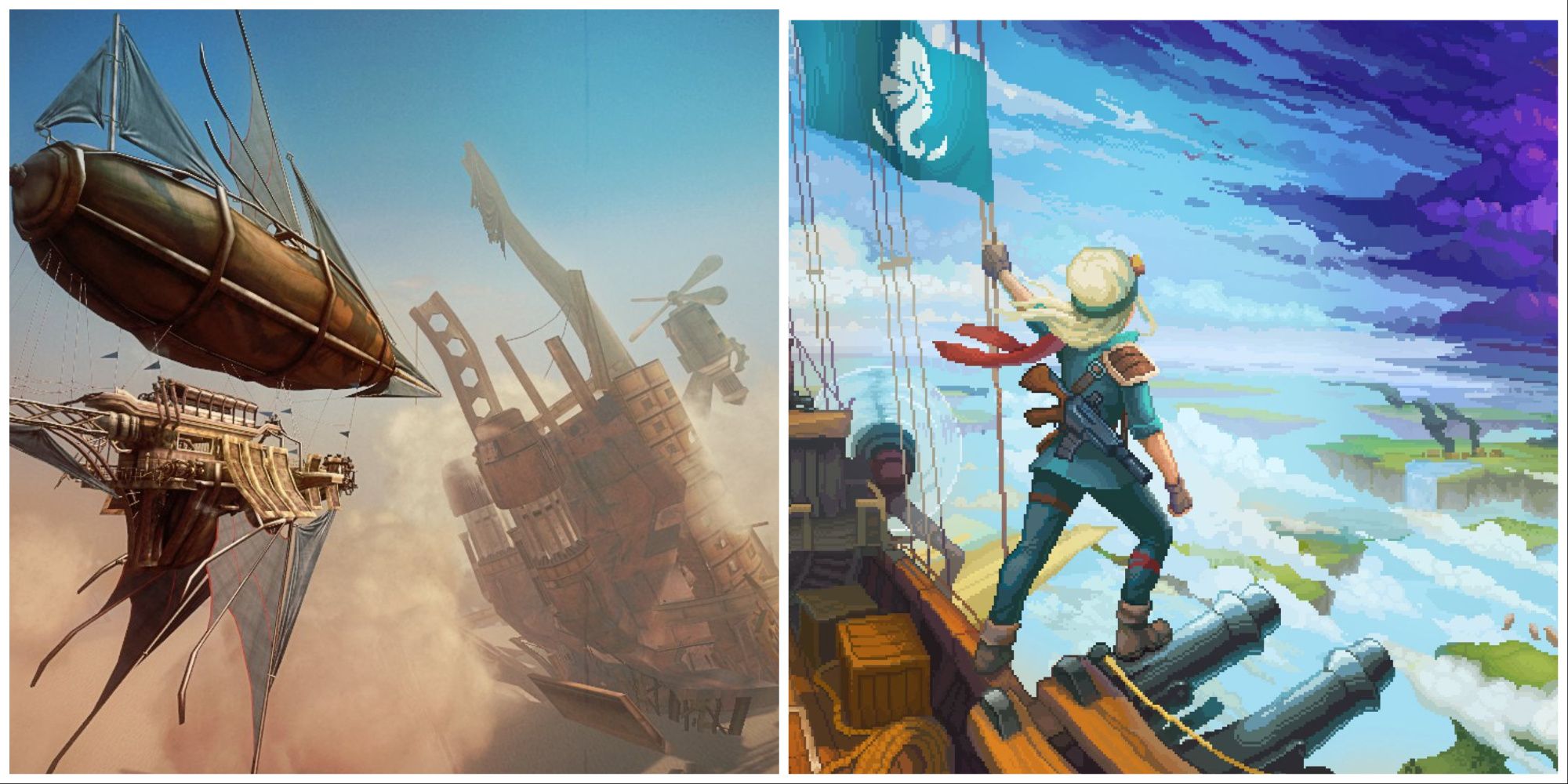The image is a detailed, two-panel computer graphic artwork. The left panel depicts a chaotic aerial battle scene above a castle, featuring various brown, blimp-like airships with sails and weapons. These dirigible vessels resemble spaceships, some equipped with daggers, and others resembling helicopters or circular bombs, all engaging in combat amid the sky. The castle below is significantly damaged, with parts of it crumbling, indicating the intensity of the battle. There is also a windmill visible on top of the castle, contributing to the scene’s drama.

In the right panel, an individual dressed in a turquoise outfit with a gun slung over their shoulder stands on the deck of a steam-powered, brown ship. This person, possibly a captain or a kid, is holding onto a flagpole that bears a turquoise flag with a white seahorse emblem. The character’s back is towards the viewer as they stare into the distance. Behind them, ominous storm clouds loom, and far off in the horizon lies a distant land with a mix of green terrain and grayish beaches, suggesting their destination or the next battlefield.